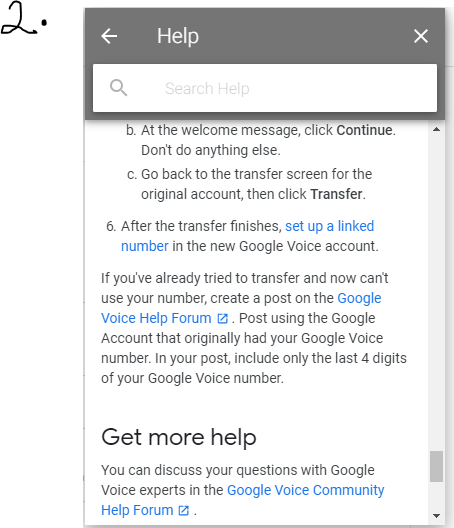A step-by-step guide on transferring your Google Voice number, presented within a well-structured interface.

At the top, the black numeral "2." followed by a grey shading, sets the stage for this guide, with a primarily white background throughout. To the left, a white arrow points backward, signifying navigation, next to a help option. On the right, a white 'X' allows for closing the guide.

Below, a white rectangle with a grey magnifying glass icon houses the text "search help" in light grey. The detailed instructions are as follows:

**B.** At the welcome message, click "Continue." Do not perform any other actions.

**C.** Navigate back to the transfer screen of the original content account and select "Transfer."

**6.** Once the transfer completes, click on “Set up a linked number” in blue, within your Google Voice account.

If you encounter issues with the number transfer:

- Create a post on the "Google Voice help forum" (linked in blue), specifying that you couldn’t use your number.
- Make the post using the original Google account associated with your Google Voice number and include only the last four digits of your number.

Lastly, for additional assistance, consult the "Google Voice community help forum" (linked in blue) to discuss questions with Google Voice experts.